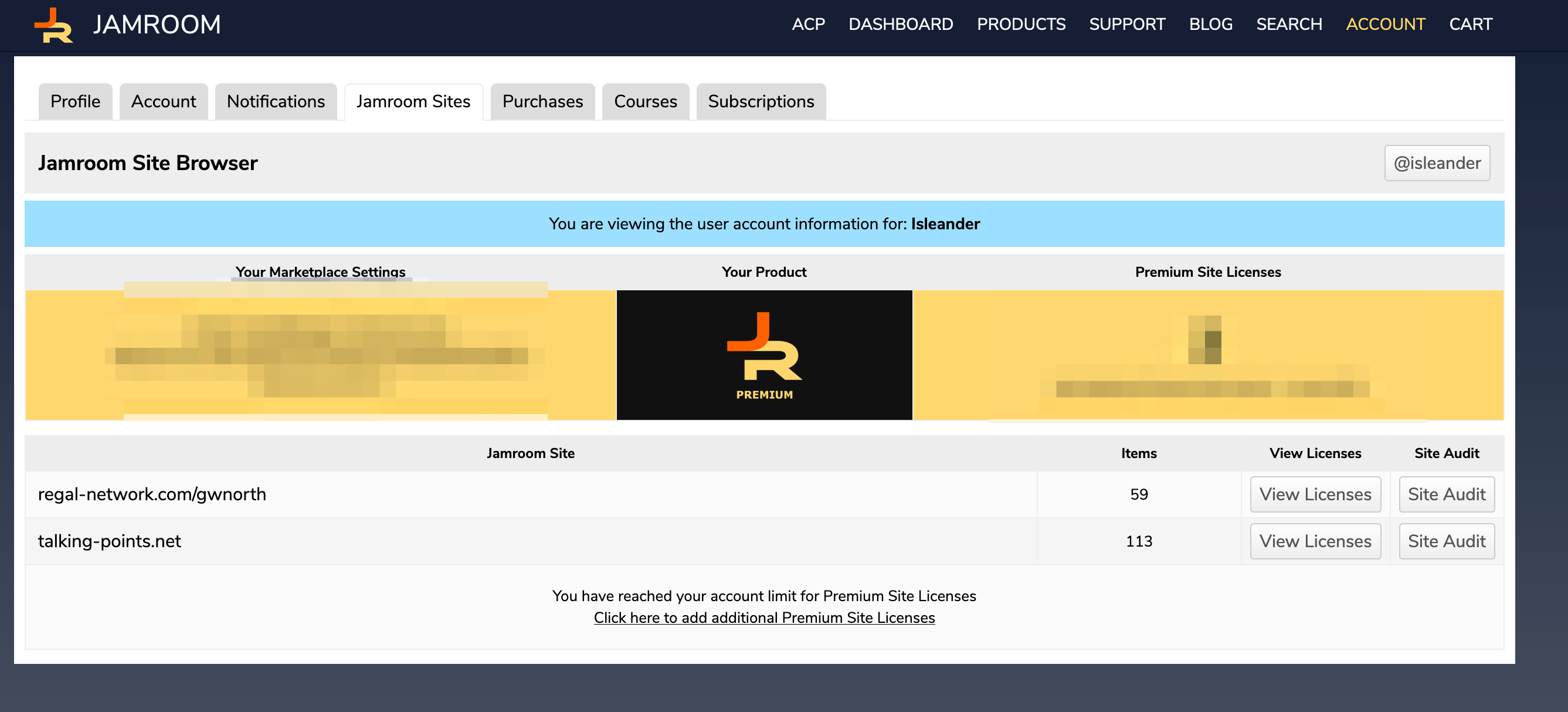A web interface is displayed within a navy blue border, suggesting it might be an app or a website. In the upper left-hand corner, an orange "J" is positioned diagonally over a yellow "R," accompanied by the text "Jam Room" in white. The header features a white menu bar with categories labeled ECP, Dashboard, Products, Support, Blog, Search, Account, and Cart. The "Account" category is highlighted in yellow, indicating it's the active page. Below this, options listed include Profile, Account, Notification, Jam Room Sites, Purchases, Courses, and Subscriptions, with "Jam Room Sites" selected.

The main content section is titled "Jam Room Site Browser" at "ISLEANDER," surrounded by a blue border and a note indicating the user is viewing account information for "Icelander." Blurred out sections read "Store Market Settings" and "JR Premium" under "Your Product." The interface lists "RegalNetwork.com/GWNorth" with 59 items, and "TalkingPoints.net" with 113 items, both of which have clickable links to view licenses and site audits. A notification states, "You have reached your account limit with Premium Licenses," with a prompt to click for adding Premium Site Licenses.